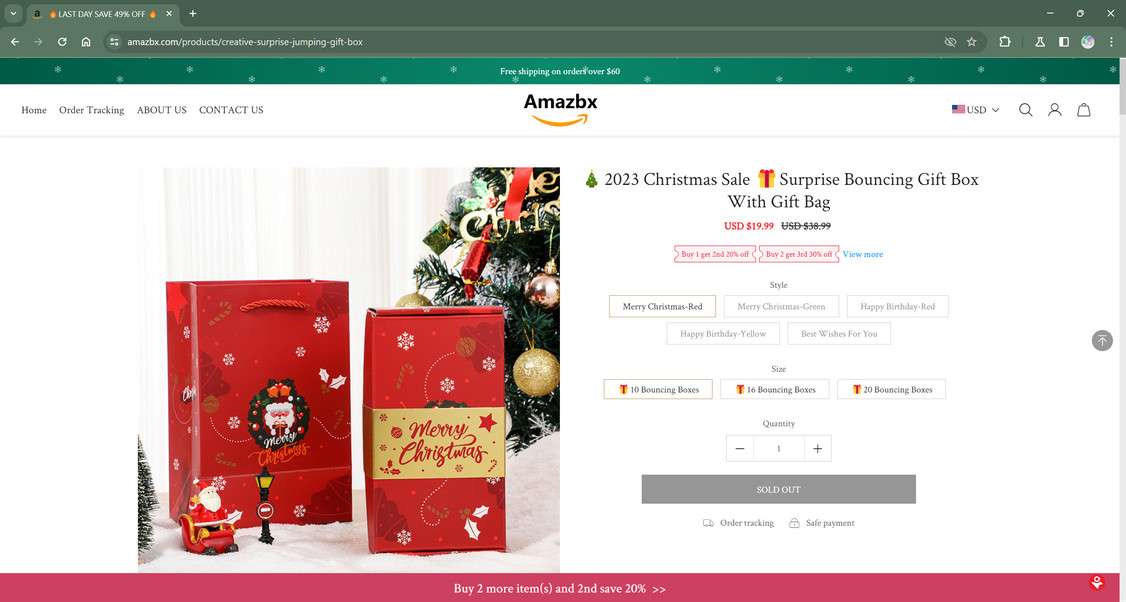The image displays an Amazon-like screen featuring a prominent banner that highlights a "Last Day Save 49%" offer. At the top center of the screen, an erroneously labeled "AMAZBX" logo is positioned, flanked by navigation options: Home, Online Tracking, About Us, or Contact Us. Towards the right side of the header, there are icons for USD currency, a search bar, a user profile, and a notification bell.

Beneath the main navigation, a vibrant announcement reads "2023 Christmas Sale," alongside a playful bouncing gift box graphic. The highlighted product is a "Surprise Bouncing Gift Box with Gift Tip Bag," priced at USD $19.99. Available festive variations include "Merry Christmas Red," "Merry Christmas Green," "Happy Birthday Red," "Happy Birthday Yellow," and "Best Wishes for You." However, all items are marked as sold out and displayed in gray.

At the bottom of the screen, a striking red bar urges customers to "Buy two more items and save 20%." Additionally, it reassures users with notes on online tracking and safe payment options. The overall scene conveys a high-urgency, festive shopping environment with a prominent emphasis on limited-time deals and product availability.